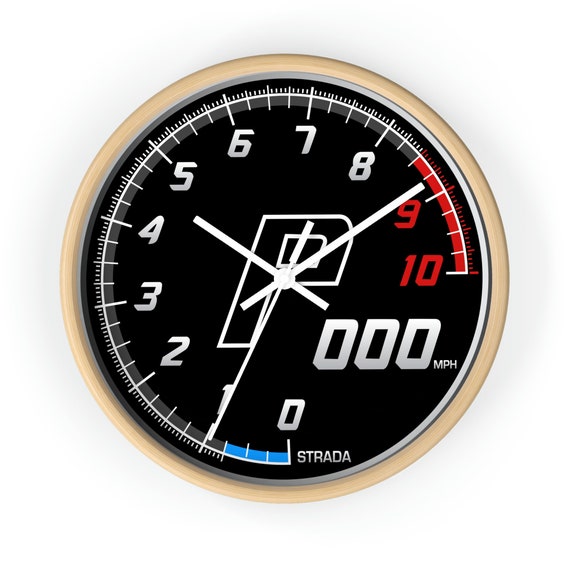The image displays a unique device resembling both a speedometer and a watch. It features a circular gauge marked from 0 to 10 in a clockwise direction, with the 0 positioned at the bottom. The area between 8.5 and 10 is highlighted in red, indicating a critical range. Notably, there are three small blue dots next to the 0, each separated by three dashes, with a similar pattern of black dots between other numbers, turning red again near the 9 and through to the 10. 

In the center of the gauge is a prominent "P," possibly denoting the brand or type of device. The gauge also includes three hands: a small hand positioned between the 4 and 5, a large hand set on the 9, and another hand pointing at the 1, mimicking the hands of a clock. Additionally, the gauge displays "strada" at the bottom and "000 miles per hour" in the bottom right corner. This device could be interpreted as a specialized speedometer, possibly used by runners or other athletes, combining elements of a clock without adhering to the traditional 1 to 12 hour markings.